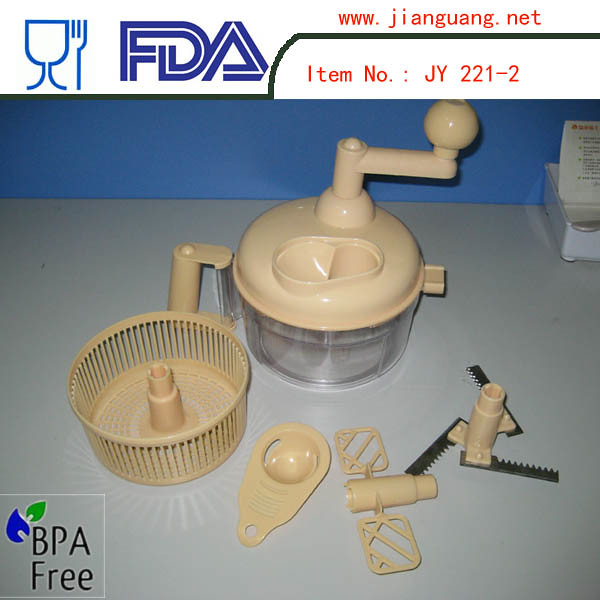This image depicts a disassembled kitchen tool, likely a manual food processor, arranged on a white countertop with a blue wall in the background. In the upper left corner, there's a blue illustration of a wine glass and fork alongside the FDA logo. The top right corner features the website "www.jiangguang.net" in red, accompanied by the item number "JY221-2" in red beneath it. The device itself consists of a cream-colored container with a clear circular base, a lid equipped with a spin handle for manually rotating the gears and blades, and a vented basket suitable for use as a salad spinner or strainer. Additional accessories, such as a detached blade, a stirring device, and a measuring tool, lie on the counter. In the lower left corner, the text "BPA-free" appears in black, surrounded by a blue and green border. The setup is complemented by a piece of paper with indistinguishable text, positioned on a stand.